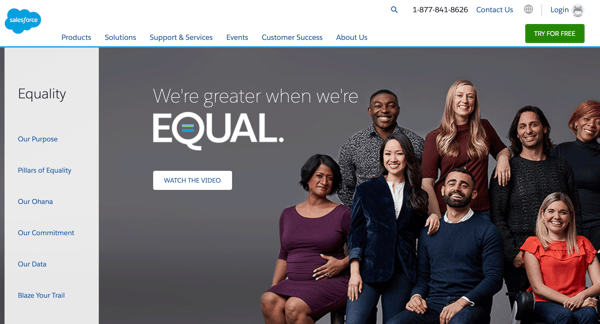The image depicts a webpage with a clean, professional layout, primarily associated with Salesforce. In the upper left corner, the Salesforce logo stands out against a blue background. Running horizontally across the top of the page, a navigation bar lists several links: Products, Solutions, Support and Services, Events, Customer Service, and About Us. On the upper right corner, there are additional contact options, including a phone number, a 'Contact Us' link, and a 'Login' button. Below these, there's a green 'Try for Free' button.

The left-hand column of the page is dedicated to various topics under the theme of Equality. The listed topics include Equality, Our Purpose, Pillars of Equality, Our Ohana, Our Commitment, Our Data, and Blazer Trail. The main content area, occupying the majority of the page, features a large, vibrant photo of a diverse group of eight people with the slogan “We're Greater When We're Equal.” The word "EQUAL" is prominently displayed in all capital letters, with two horizontal lines inside the "Q," one in a light green or light blue hue and the other in a medium blue. Beneath this bold message is a link prompting users to "Watch the Video."

The group photo showcases a diverse assembly of eight individuals. On the far left, a woman seated in a purple dress begins the lineup. Next to her, a man in a gray sweater stands in the background while a woman in a dark suit stands and smiles in the foreground. Moving right, a woman with long blonde hair wearing a maroon top stands behind a broadly smiling man in a blue long-sleeve shirt who is sitting. Continuing right, a man in a sweater stands in the background beside a seated woman with long blonde hair, dressed in an orange top. Finally, on the far right, a woman stands, donning a black top.

The image and accompanying text collectively convey a strong message about equality and inclusivity within the Salesforce community.